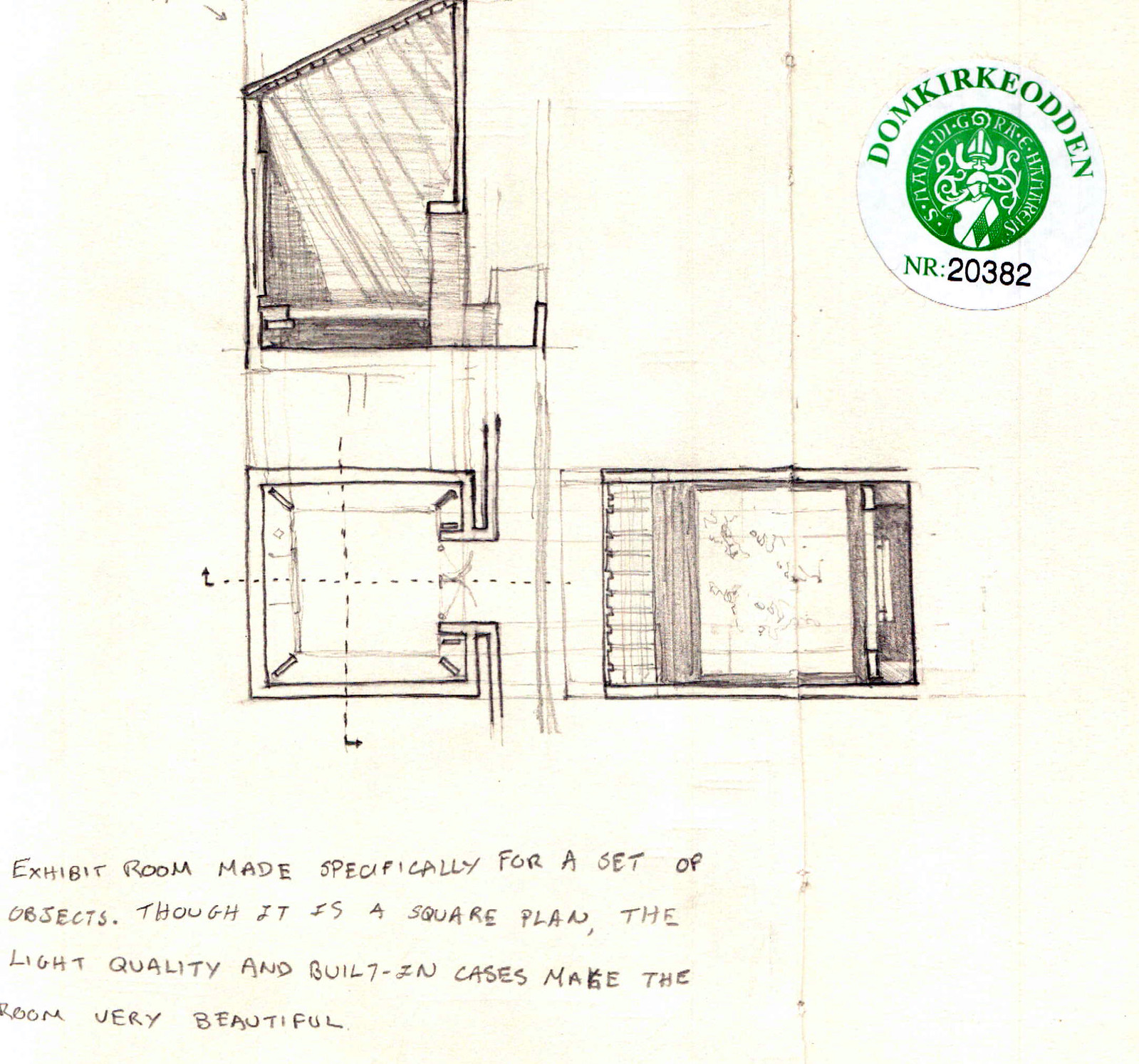This image depicts a detailed architectural blueprint, showcasing three rooms drawn in pencil or pen. In the upper right-hand corner, there's a prominent white circle featuring the name "Dom Kirk Eoden" in green letters, accompanied by the firm's green and white circular logo. Below these identifiers is the inscription "NR 20382." The blueprint appears to illustrate a square room with a door on the right, a more rectangular room immediately to the right, and another rectangular room above with a slanted roof. In the lower left-hand corner, there's a handwritten or printed note stating, “Exhibit Room, made specifically for a set of objects. Though it is a square plan, the light quality and built-in cases make the room very beautiful.” The detailed notation emphasizes the aesthetic quality imparted by the lighting and built-in display cases within the exhibit room.